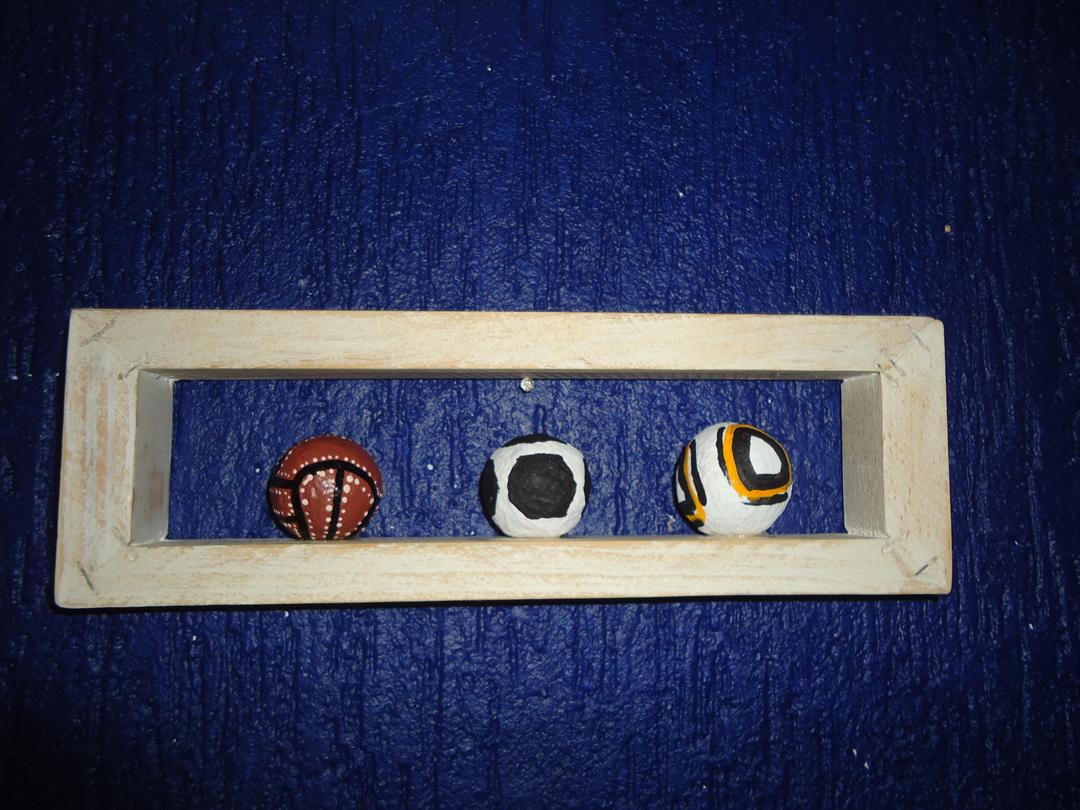In a dimly lit room where the edges fade into blackness, a dark blue, rough-textured plaster wall serves as the backdrop for a distinctive display. Mounted on this wall is a long, rectangular wooden frame with a rustic, rough-hewn appearance. Suspended within the frame are three uniquely painted balls, evenly spaced.

The ball on the left is a reddish-brown color adorned with black lines and white spots. It catches the eye with its intricate pattern. The central ball is immediately recognizable as a classic soccer ball, predominantly white with striking black hexagons. On the right, a primarily white ball features intriguing black and orange circles resembling disembodied eyes, adding an element of mystery to the arrangement. This composition within the wooden frame against the textured blue wall creates a visually rich and detailed focal point in the otherwise shadowy environment.